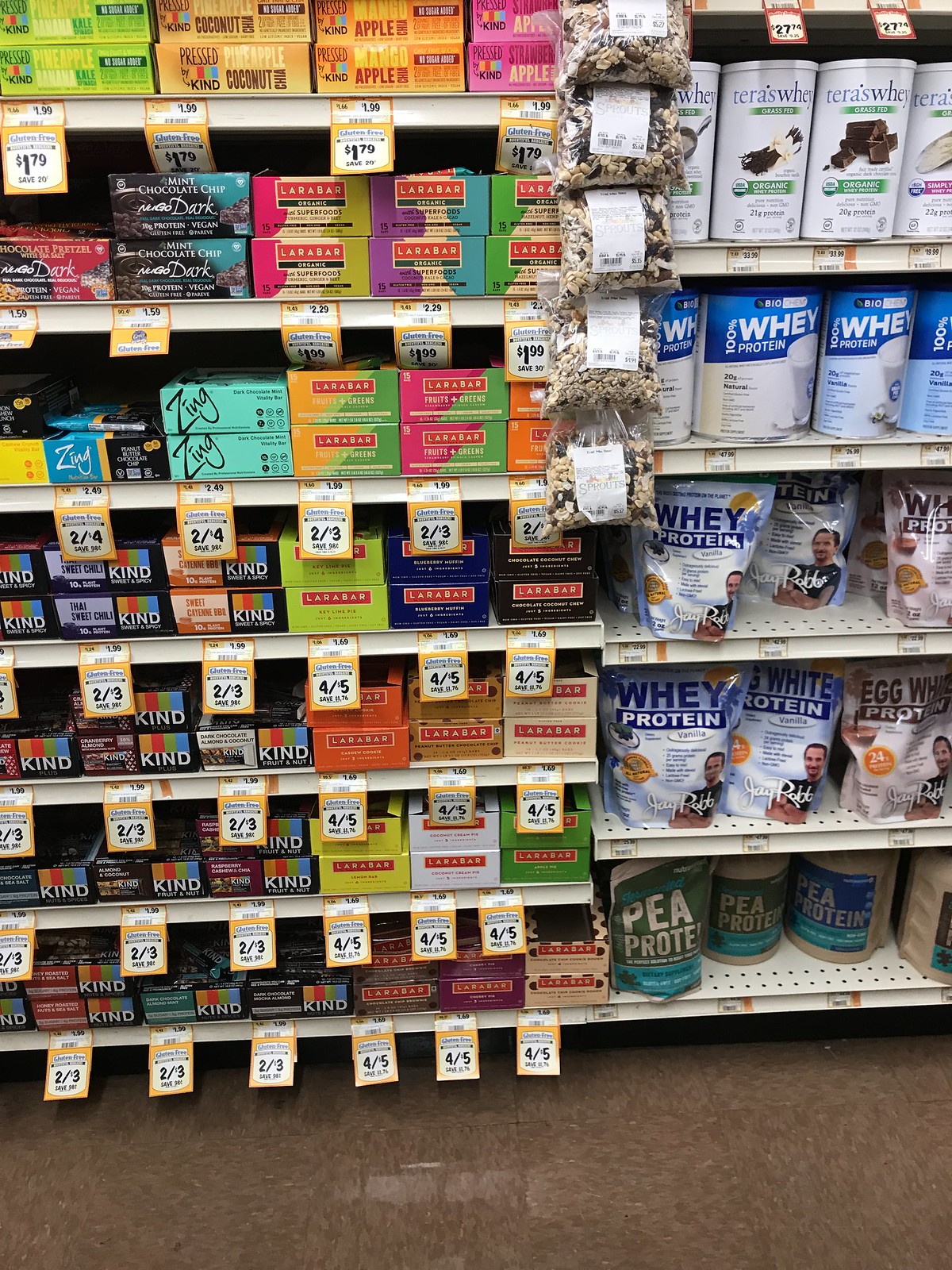The photograph captures a well-organized section of a grocery store's aisle, showcasing a vibrant display of protein and nut bars. The shelves are meticulously stocked with an extensive variety of bars from renowned brands such as LÄRABAR and KIND, among others. The assortment features an array of flavors, creating a visually striking tapestry of colors that almost resembles a tie-dye pattern. Promotional tags on the shelves indicate various sales, with offers like "two for $3" and "four for $5." On the right side of the image, canisters of protein powder, including whey and pea protein variants, are prominently displayed. Hanging from the shelves, there are also packets of trail mix, adding to the diverse selection available in this section. The image captures the bustling, colorful essence of a grocery store aisle dedicated to health-conscious and high-protein snack options.